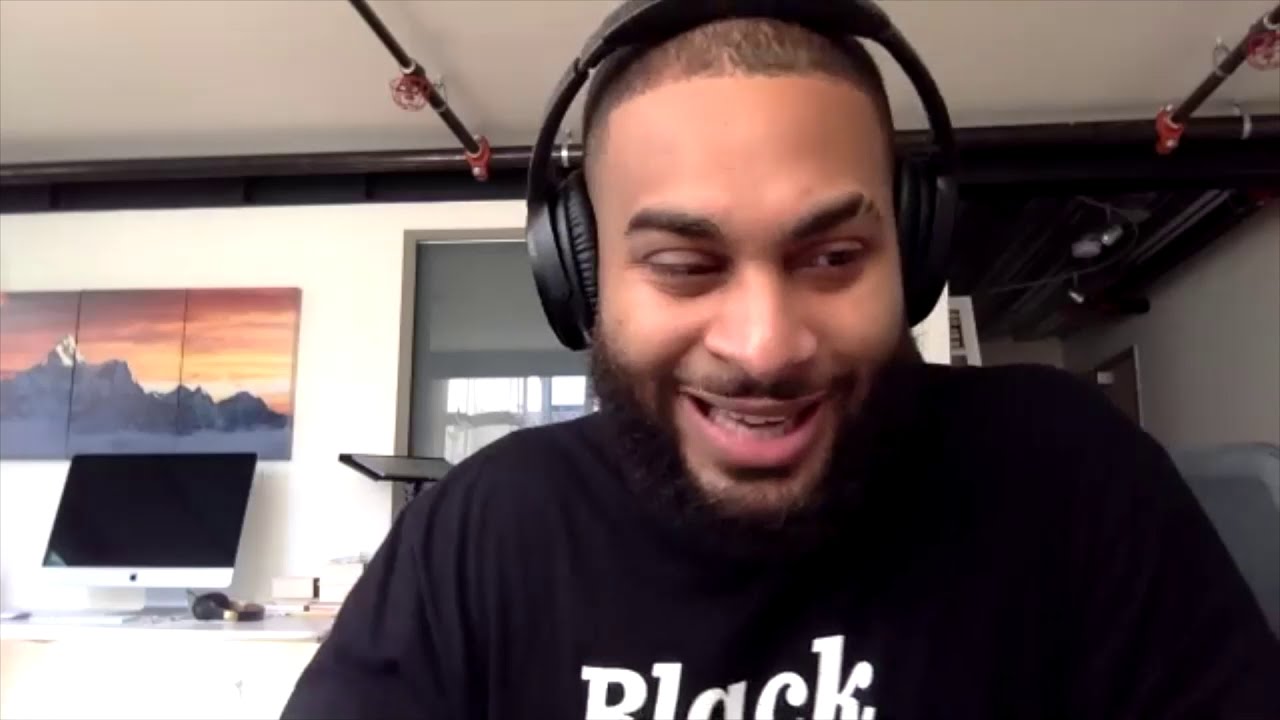The image captures a young Black man with a neatly trimmed beard and a stylish fade, wearing black headphones and a black t-shirt with partially visible white text that appears to say "black." He's smiling broadly, seemingly enjoying himself, perhaps immersed in music or engaging in a joyful conversation. The setting suggests a media or audio production studio, characterized by an Apple monitor and various pieces of equipment on a white desk to his left. Above the monitor hangs a striking three-panel painting depicting a mountain landscape under a vibrant sunset sky. The room's walls are pale yellow, and a large window with a partially rolled-up black and gray shade, as well as curtains, is situated behind him to the left. The ceiling features white paint with pipes and rods, some with red fittings, running across it. The overall ambiance is one of creative joy and a professional yet relaxed environment.